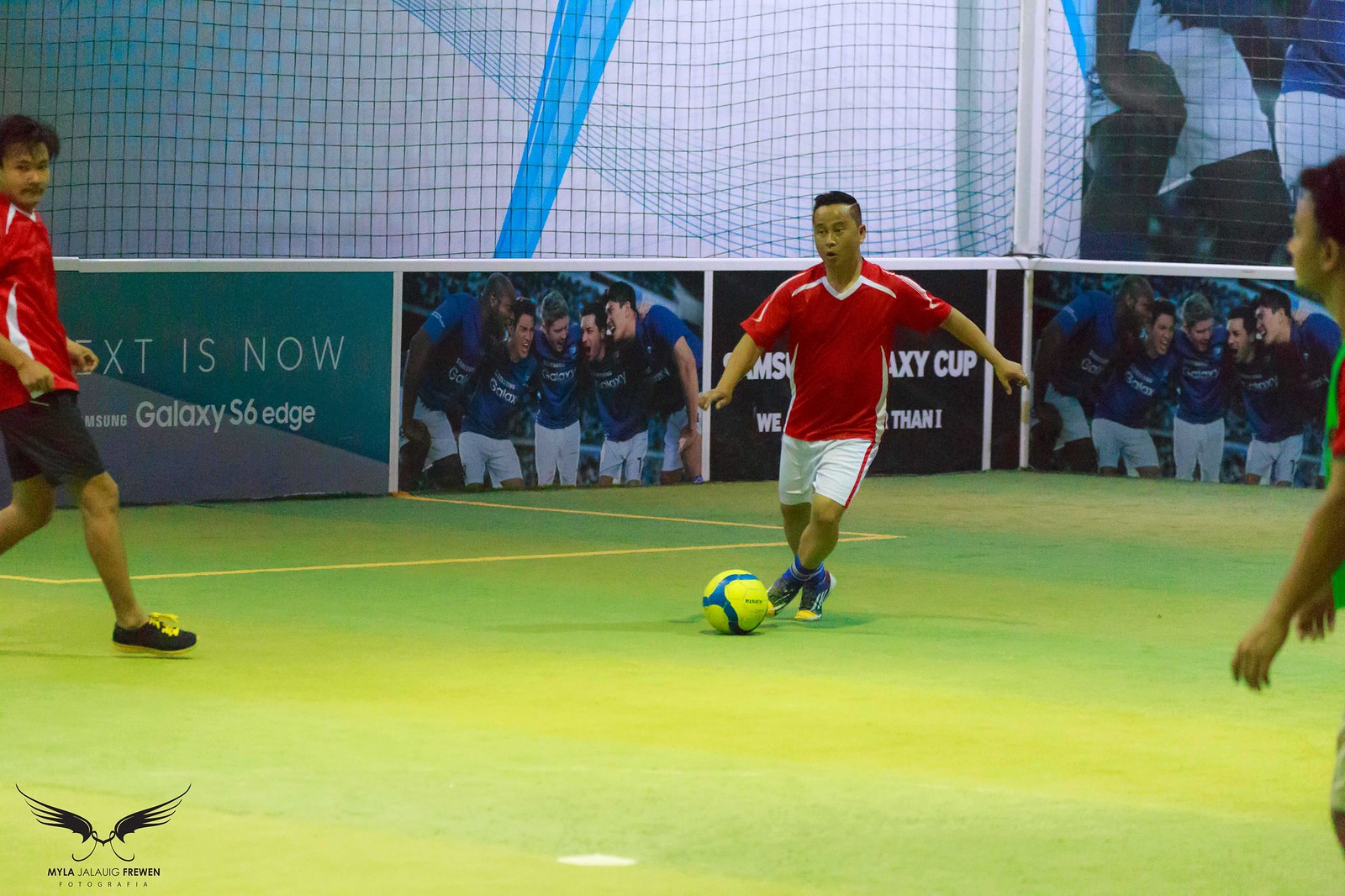This is a horizontally aligned rectangular image capturing live action during an indoor soccer game on a lime green turf. In the center, a soccer player with short black hair, dressed in a red and white jersey and white shorts with red stripes, is about to kick a blue and yellow soccer ball. His mouth is open in an 'O', arms out by his sides, legs crossed, showing movement. He wears blue and yellow shoes. In the far left of the image, another player in the same red jersey but with black shorts and black and yellow shoes is visible, looking towards the camera. On the right, there's a player in a red top with something green over it. The background features a large net and a border wall adorned with various banners, including those for 'Galaxy SX Edge' and the 'Samsung Galaxy Cup'. Some banners depict a group of teammates huddled together. In the lower left-hand corner, there's a small logo with black wings and the text "Myla Jalog Bruen, Toto Graupia," although the text is hard to read. The scene suggests a casual game without goalies or referees.